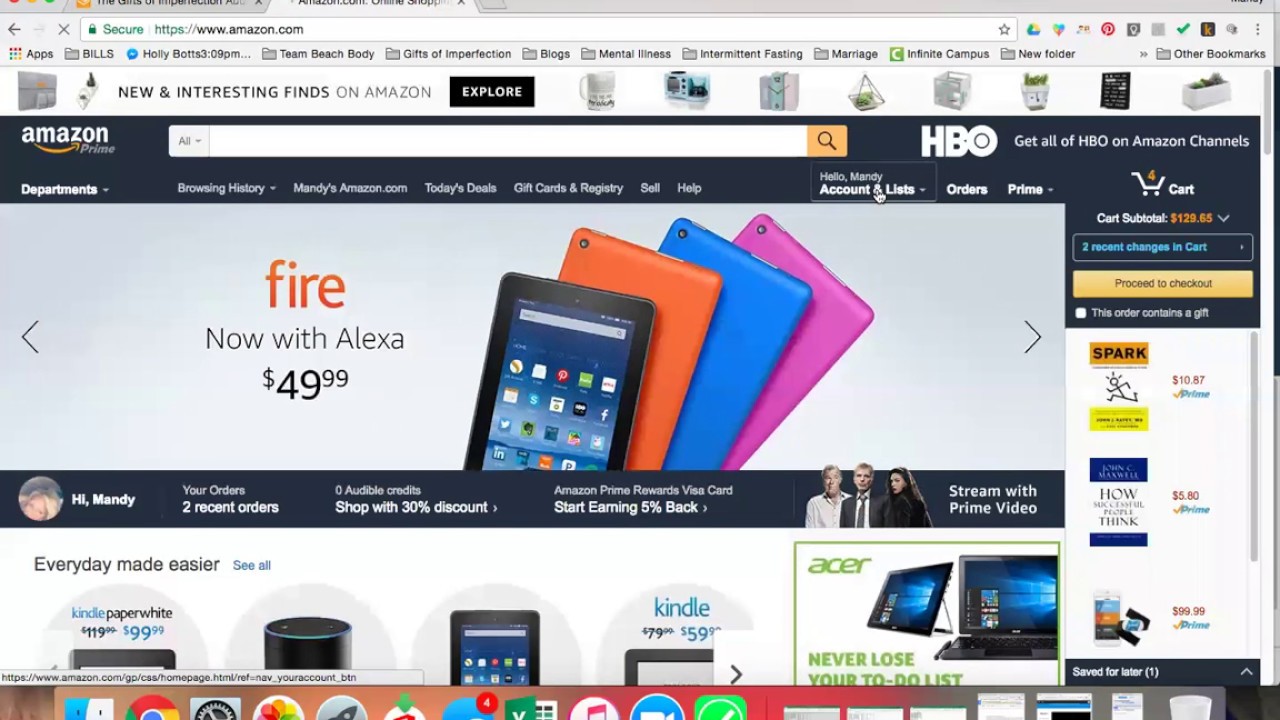A screenshot of the Amazon.com homepage on a desktop displays the main promotional banner for the Amazon Fire tablet with Alexa, priced attractively at $50. The user is signed in, as indicated by the greeting "Hi Mandy.” Various account details are visible, such as recent orders and zero Audible credits, along with an incentive to start earning 5% cash back.

The top right corner of the page shows four items in Mandy’s cart, with a subtotal of $129.65 and a "Proceed to checkout" button directly below. Other visible items on the page include multiple tablets, an Alexa speaker, an ad for an Acer laptop, and a book, albeit with text too small to read. The page retains Amazon's characteristically dense and busy user interface.

An HBO advertisement, promoting access to HBO through Amazon Channels, is also present in the top right corner, suggesting this might be an inclusion with Amazon Prime.